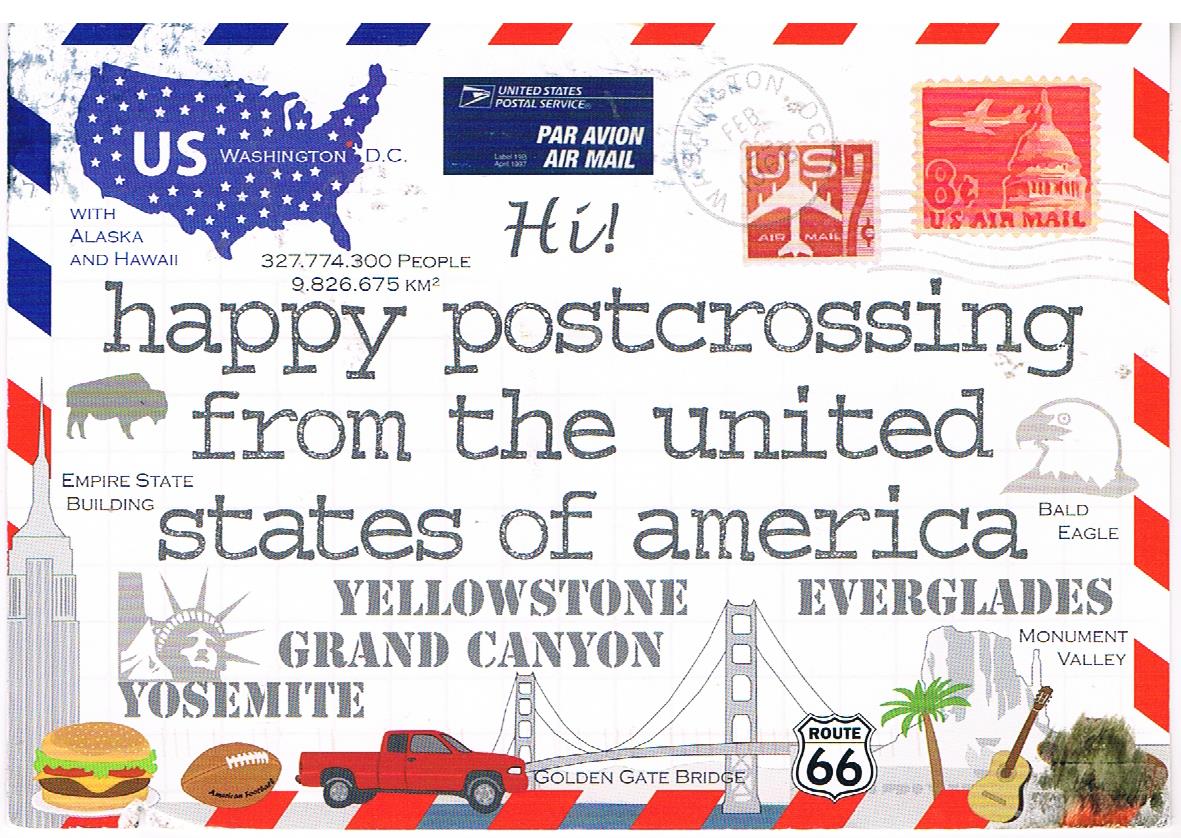This image depicts a vibrant and busy postcard adorned with iconic American symbols and landmarks. The postcard features an assortment of graphics, including the Statue of Liberty, Empire State Building, Monument Valley, a bald eagle, and the Golden Gate Bridge, all clearly labeled. Additionally, it showcases a map of the United States in the top left, marked with Washington, D.C. The card is bordered by a distinctive red and blue stripe, reminiscent of traditional airmail design.

In the center of the postcard, the text reads, "Hi, happy post crossing from the United States of America," accompanied by bold mentions of Yellowstone, Grand Canyon, Yosemite, and Everglades. The lower section of the postcard highlights American cultural icons, such as a cartoon hamburger, football, red pickup truck, and a sign for Route 66, along with a palm tree and an acoustic guitar. The top right corner features two U.S. stamps and the phrase "United States Postal Service, airmail," indicating it has been processed through the mail. Overall, the postcard is a nostalgic celebration of American imagery and landmarks.